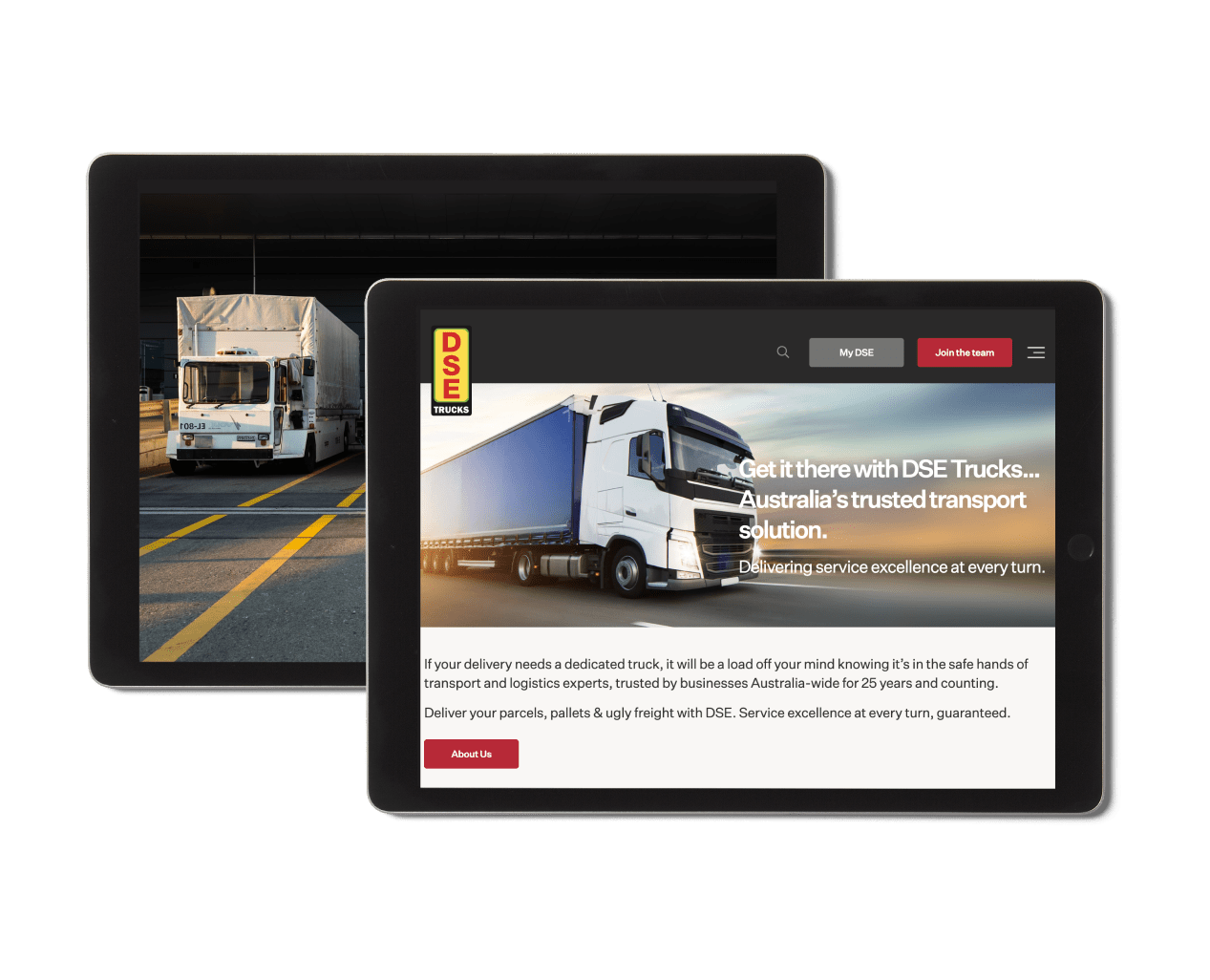The provided image is comprised of two simulated tablet screenshots. Each screenshot features distinct content framed by black, rounded-corner borders and grey edges, mimicking the appearance of actual tablets.

In the screenshot on the left, a truck is prominently displayed, parked beside dual yellow lines. The setting includes a black wall adorned with horizontal bars, a sunlit road, and overall urban surroundings.

The right screenshot is detailed with multiple elements. At the top, there's a black bar containing various icons and text boxes. On the left side of this bar, a rectangular icon displays "DSE" in red on a yellow background. Below this is a black strip with the word "Truck" written in white. Further right, a search icon is followed by a grey box labeled "my DSE" in white, a red box stating "Join the Team" also in white, and an icon with three horizontal lines.

The main visual element is an image of a white-fronted truck with blue sides, driving along a road. This scene is backdropped by a hazy, twilight skyline, blending hues of yellow, blue, and scattered clouds. Superimposed over this image is large white text reading: "Get there with DSE Trucks... Australia's trusted transport solution, delivering service excellence at every turn." 

Below this header, a block of black text on a white background explains the company's services, emphasizing their 25 years of expertise in providing safe, reliable transport and logistics solutions across Australia. Key services mentioned include parcel, pallet, and "ugly freight" delivery, emphasizing their guarantee of service excellence. At the bottom left, a red box with the word "About" in white concludes the description.